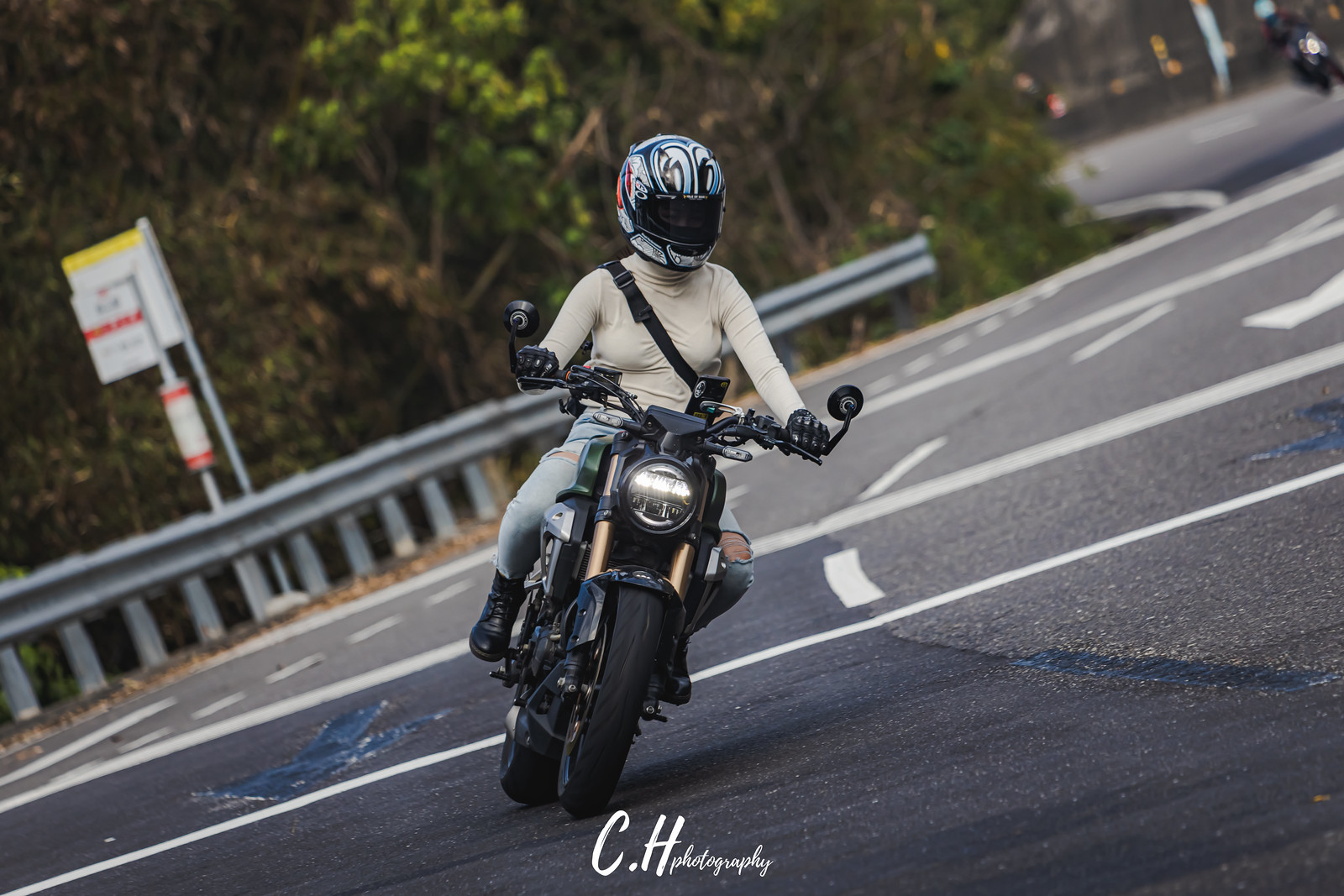A vibrant photograph captures a woman in the midst of a turn on her green and silver motorcycle, leaning slightly to the right as she navigates the gray asphalt roadway, which is marked with multiple lines indicating traffic crossings, lanes, and sides of the road. The motorcycle, featuring a large, round, white headlight, black handles, black wheels, and gold-colored suspension bars, appears powerful and dynamic against the urban backdrop. The woman is dressed in a tight-fitting long-sleeve white turtleneck sweater, blue jeans with torn knee sections, and black gloves, her look completed by black boots. She is gripping the handlebars firmly, her helmet adorned with blue, black, and white stripes, and a dark opaque visor shielding her eyes and nose. Partially visible is a black strap from her shoulder bag slung across her chest. Behind her, the road curves to the left, bordered by tall shrubs, with another motorcyclist faintly visible in the distance. The photograph is watermarked at the bottom with "CH Photography" in white text.